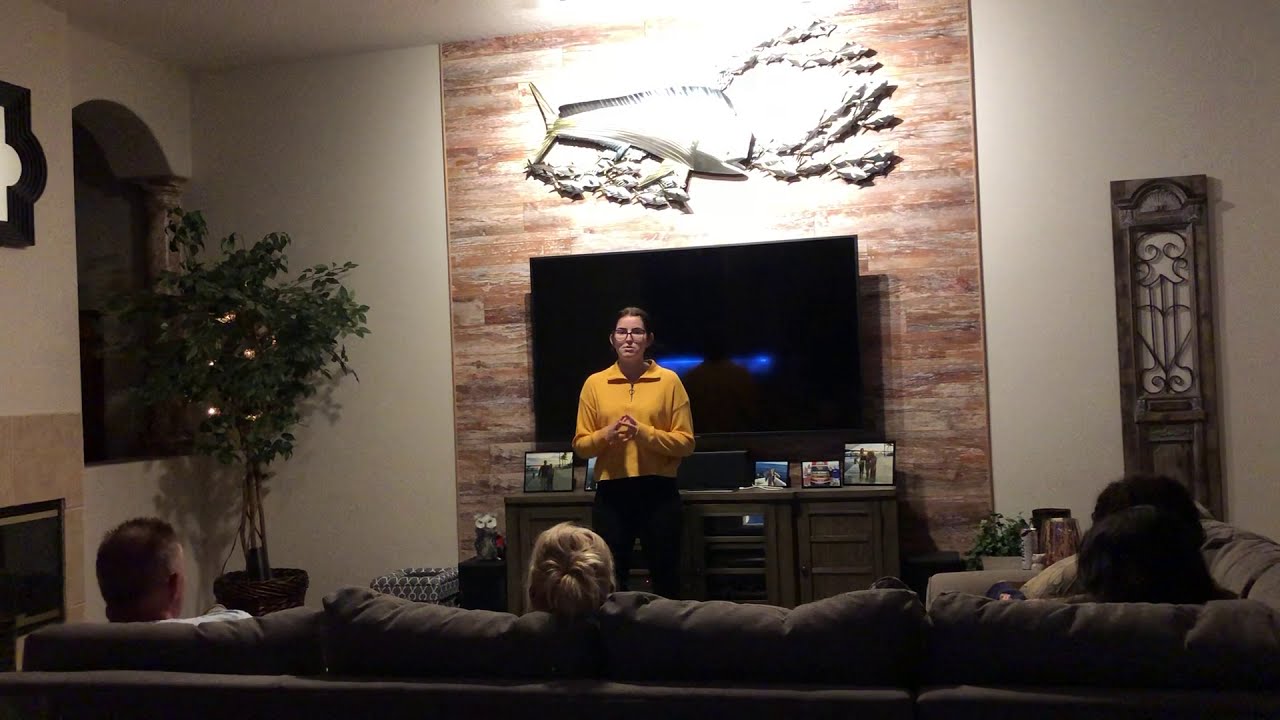The image captures an indoor scene, likely in a living room decorated with various items. Four people are seated on a dark gray couch with only the backs of their heads visible. These include a White male with dark hair, a female with blonde hair, and two other individuals with dark hair. They are attentively facing a white person of indeterminate gender, who is standing in the center of the room. This central figure has glasses, dark brown hair, and is dressed in a yellow sweater and black pants, appearing to address the seated group seriously.

Behind the standing person, there is a TV on a brownish-gray TV stand, accompanied by several family photos. An unlit fireplace and a tall silk tree in a pot are situated to the left, contributing to the cozy ambiance of the room. The walls are off-white, and there is decorative wall art, including a whale above the TV and likely some grill work off to the right. The room is well-lit, with various hues of gray, tan, black, green, yellow, blue, and brown adding splashes of color.